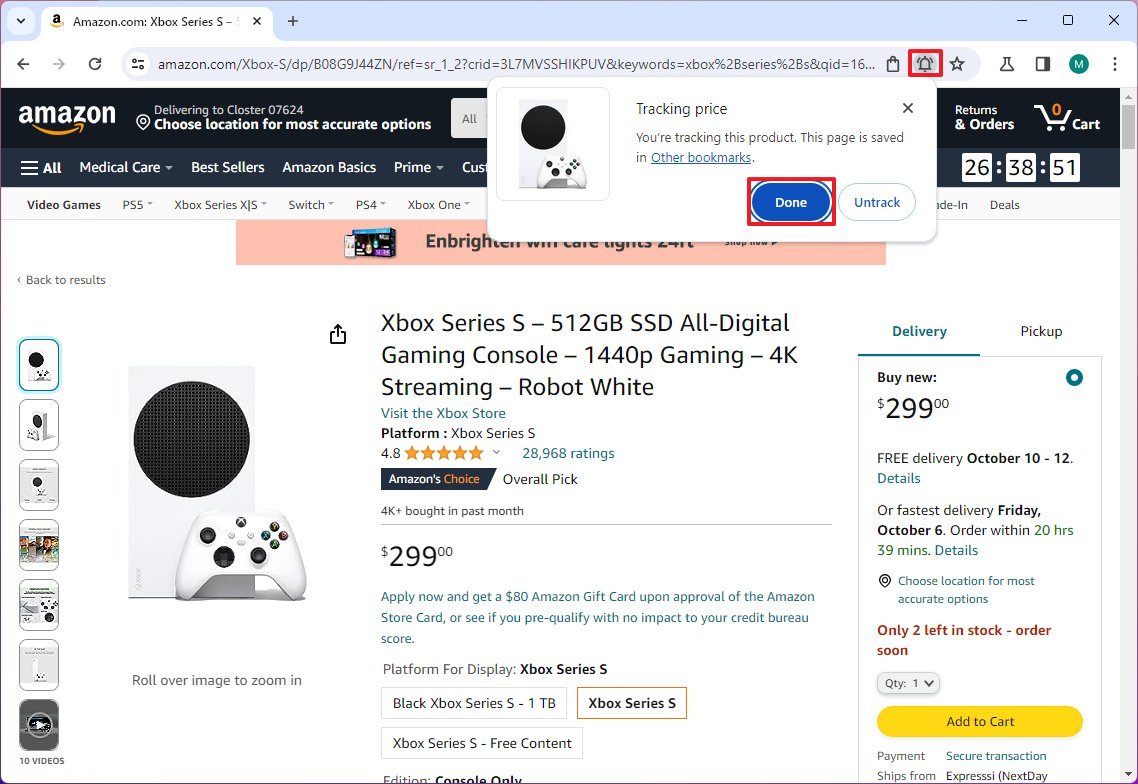The Amazon.com webpage showcases the Xbox Series S, a sleek, all-digital gaming console with a 512 GB SSD. The device, designed in a distinctive "Robot White," supports 1440p gaming and 4K streaming experiences. The console itself is compact and triangular in shape, featuring a prominent black circular vent in the center. Accompanying the console is a white controller, equipped with black buttons and joysticks. The face buttons are marked with the familiar Y, A, B, and X. This product is listed at $299.

In the upper left corner of the webpage, the iconic Amazon logo with its characteristic orange arrow is visible. A sidebar indicates the user is tracking this item for price changes. Additionally, a blue button labeled "Done," highlighted in red, appears, suggesting the page is saved in the user's bookmarks.